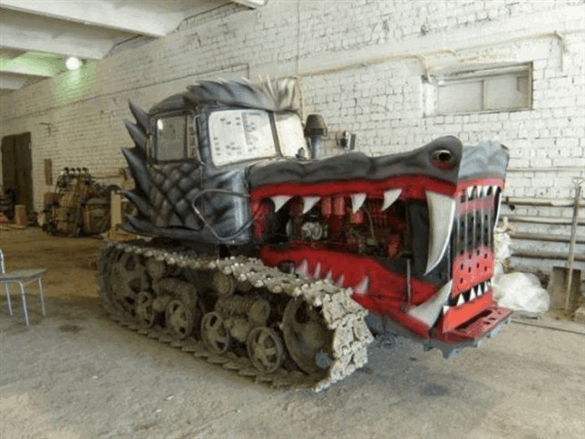This photograph captures a uniquely designed vehicle resembling both a tank and a tractor, artistically styled to mimic the ferocious appearance of a wolf. Equipped with tank-like treads instead of wheels, the main body of the vehicle is painted gray with exposed engine parts, particularly visible in its gaping red mouth filled with sharp, white teeth. The mouth resembles a snarling wolf's snout, adding a menacing flair. The cab, representing the wolf’s head, has simulated fur textures around the windows, which appear as eyes. The vehicle is parked in a white brick garage, complete with various tools on the far left wall, a light in the top left corner, and a chair near the left side on a hard concrete floor.